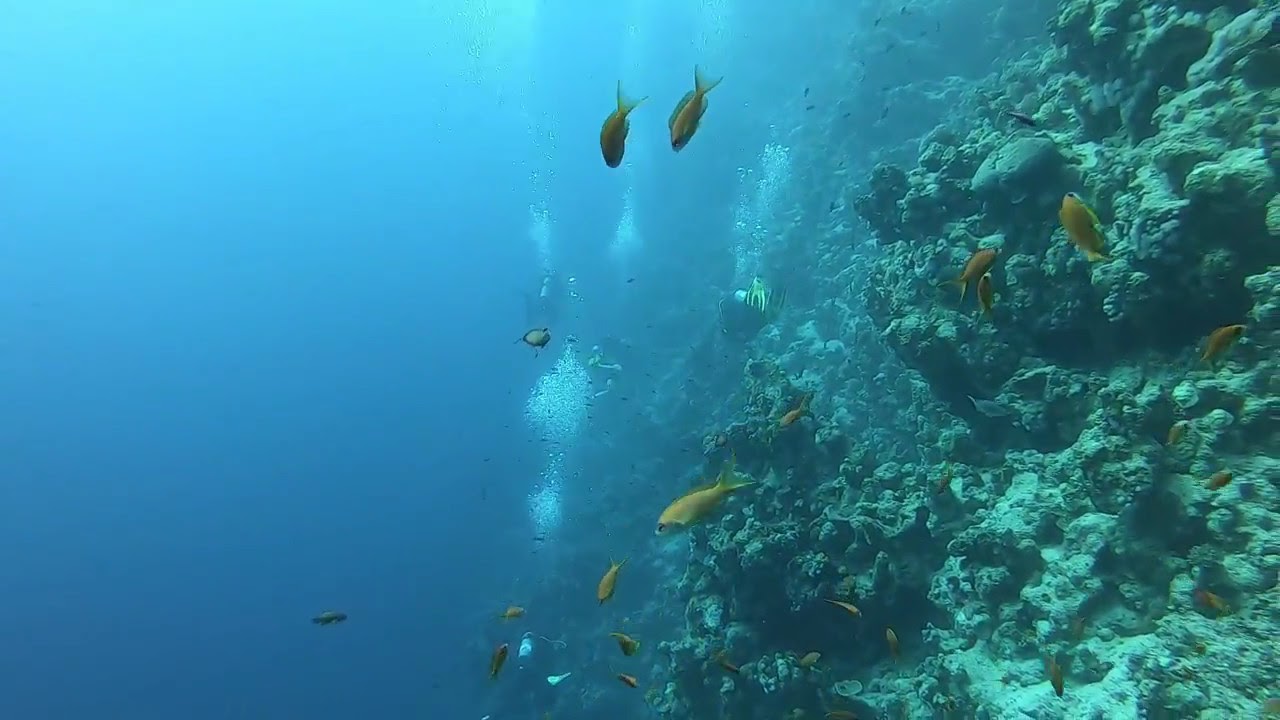This underwater photograph, likely taken through a glass tank, depicts a serene marine landscape illuminated by daylight. Dominating the right side is a sizeable, predominantly green coral reef adorned with bubbles ascending through the water. Numerous ovate, golden-brown fish with nearly transparent fins swim around the coral, accompanied by a school of bright yellow and orange fish, creating a lively aquatic scene. The left side of the image fades into the vast blue expanse of the ocean, transitioning from a lighter greenish-blue tone near the top to a deeper blue towards the bottom. Amid this tranquil blue void, the faint silhouettes of three to four scuba divers are discernible, their presence indicated by streams of air bubbles rising to the surface. Despite the murkiness, the divers' activity adds a dynamic element to the otherwise gentle underwater tableau.